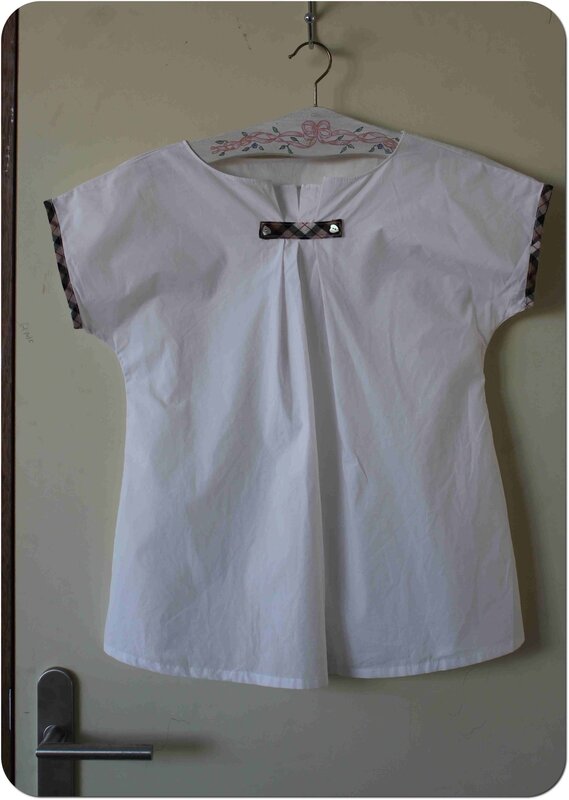The image features a woman's blouse hanging on a hanger suspended from a hook attached to what appears to be a stained, white door, as evidenced by the silver door handle at the bottom left corner and some potential writing on the wall. The blouse itself is predominantly white with a wide neckline and pleated detail at the front. It has short sleeves ending just below the armpits, each adorned with a narrow strip of trim featuring a black, white, and gray crisscross pattern. This same pattern appears in a rectangular patch at the neckline, secured by two buttons at either end. The hanger holding the blouse has a decorative ribbon design across the underside, featuring a pink flower and green leaves set against a predominantly white background, with a metal hook.